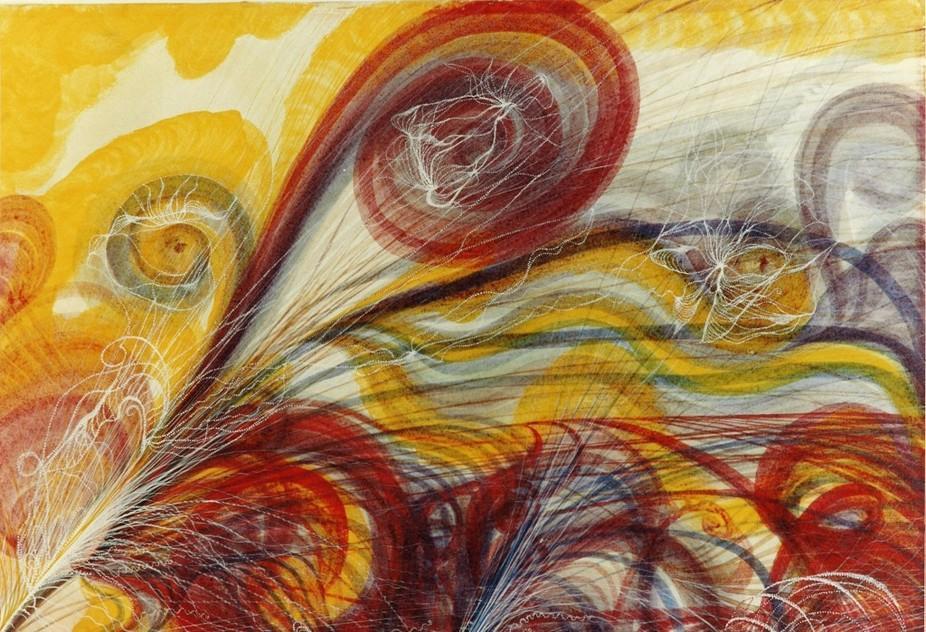This abstract mixed-media painting features a vivid interplay of colors and swirling forms that evoke the delicate texture of peacock feathers. Originating from the bottom left and lower center, the composition radiates outward with dynamic lines and spirals in shades of yellow, red, and dark blue. These lines, which increase in boldness and intensity as they move from left to right, appear to be interwoven and curling around each other in wave-like forms. The intricate spirals at the top of the painting are accentuated by red, yellow, and light blue hues. Strands of white fibers meander through the scene, adding a textured dimension that enhances the painting's abstract quality. The background is predominantly yellow, providing a luminous backdrop that contrasts with the more pronounced and vibrant spirals and lines. The bottom of the image features distinctive red strokes that circle and move horizontally toward the bottom right corner, culminating in a composition rich with movement and layered depth.